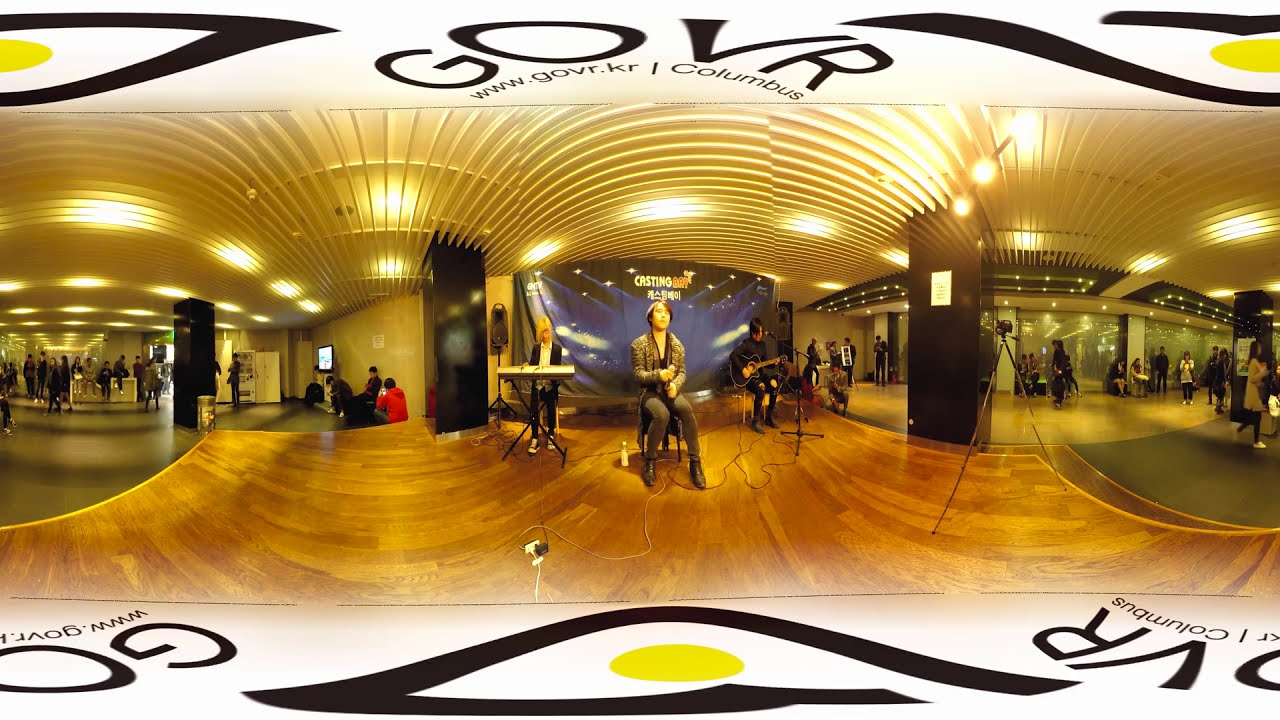In an expansive venue that resembles the hallway or corridor of a large building, a small stage is set up where a trio of young men are performing. The stage is lightly colored in shades of yellow and brown. The trio consists of a keyboardist wearing a black jacket over a white shirt on the left, a guitarist seated on the right, and a singer sitting at the front center holding a microphone. The singer is the focal point of a recording setup, with a camera positioned on an apparatus aimed at him. Surrounding the scene, several spectators wander through the corridor, some leaning against the walls, others walking about or engrossed in their phones. A sign above the musicians possibly reads "casting," hinting at a formal event or audition, while the overall atmosphere suggests a company or government-sponsored gathering.